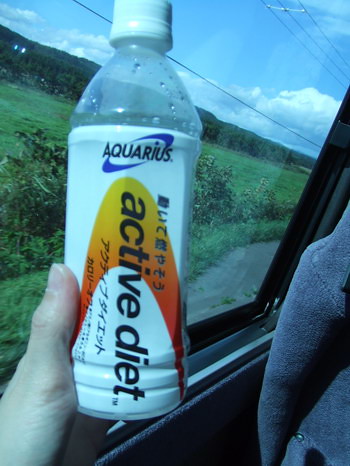This photograph captures a clear plastic sports drink bottle held by a person inside a vehicle, likely a car or possibly a train. The bottle, appearing empty, features a white label with prominent blue letters spelling 'Aquarius' and an 'Active Diet' subtitle in black. Adding a pop of color, the label includes a yellow and orange arc around the letters A, C, and T in 'Active.' Both Japanese and English texts are present on the label. The bottle is held by a white individual's left hand, with their thumb and part of their palm visible in the frame. The background glimpsed through a window includes lush greenery, with grass, bushes, and trees, along with telephone lines stretching across a partly cloudy blue sky.